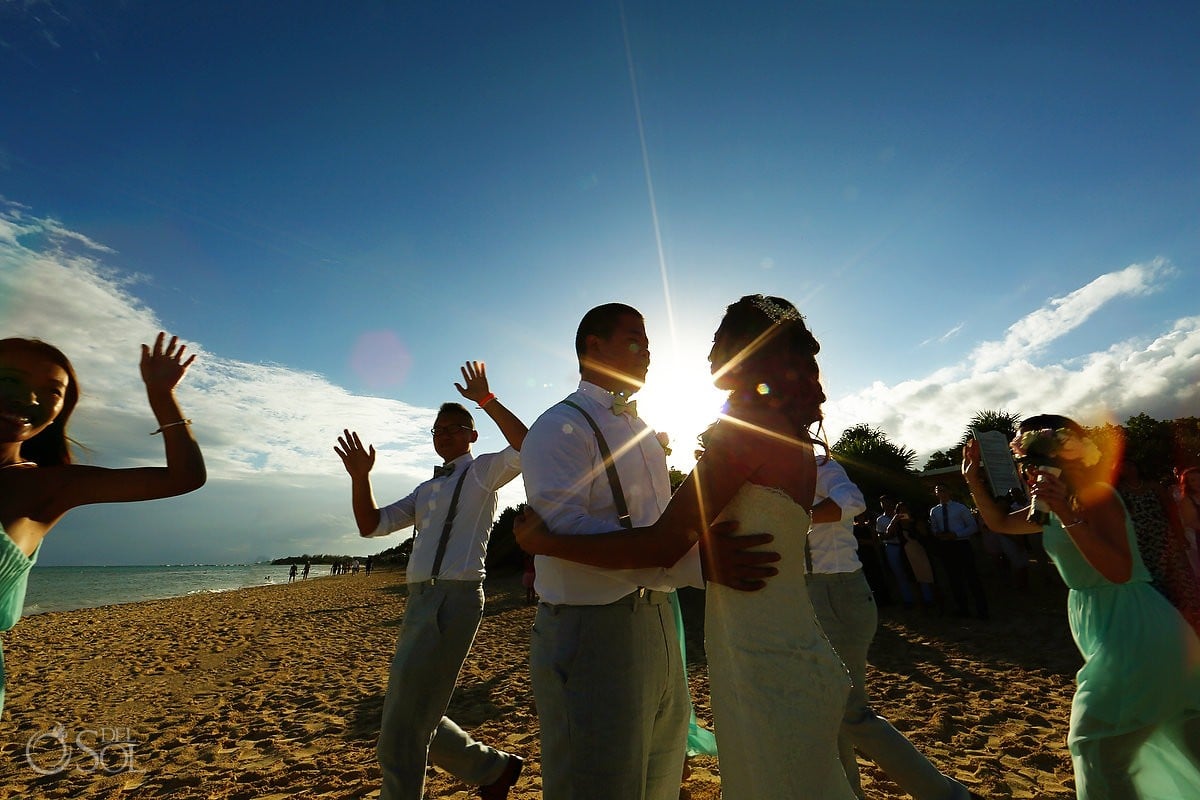In this vibrant beach wedding photograph, a black bride and groom are captured slow dancing in the center, lovingly holding each other by the waist. The bride is stunning in a strapless white wedding gown, her shoulder-length hair softly framing her face. Meanwhile, the groom complements her elegance with a white button-up shirt, grey slacks, and black suspenders. The backdrop features a sprawling, crystal blue sky dotted with a few clouds, with the radiant sun perfectly positioned between the couple, casting a warm glow and gently obscuring their faces. To the left, the calm ocean adds a serene touch to the scene, while the sandy beach extends invitingly underfoot. Encircling the couple, two men and two women—dressed in similar white button-up shirts, grey slacks, black suspenders for the men, and sea green dresses for the women, one adorned with a flower wreath in her hair—joyfully raise their hands in the air, their smiles capturing the joyous essence of the celebration. In the distance, a crowd attired in formal wear blurs into the background, enhancing the focus on the intimate, heartfelt moment shared between the bride and groom.